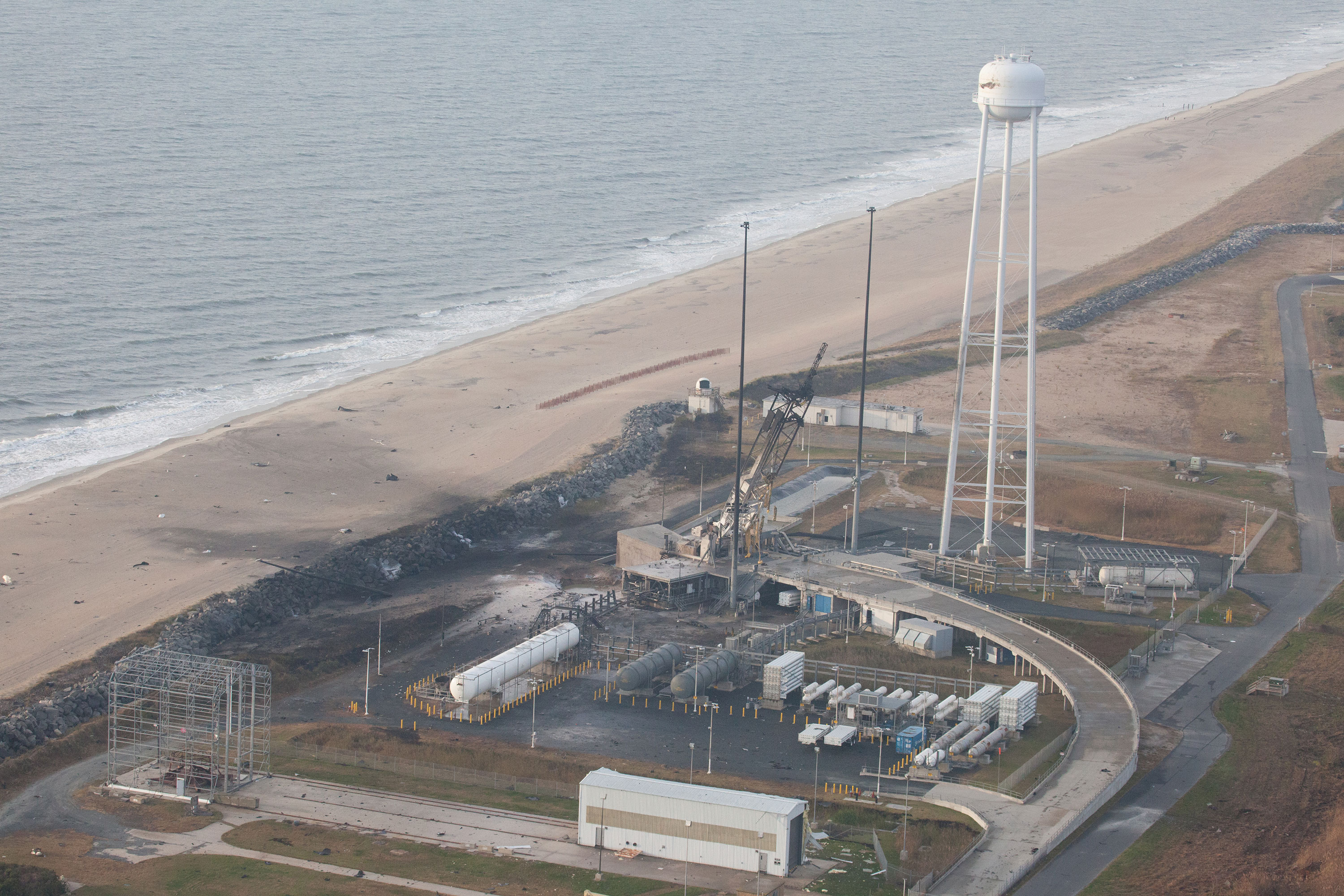This detailed aerial photograph captures an industrial plant situated adjacent to a shoreline, possibly an ocean due to the visible waves crashing against the sandy beach. Central to the plant is an exceptionally tall, white, three-legged water tower with a mostly cylindrical and slightly spherical top, overseeing the entire facility. The landscape around the plant is barren and muted in color, with patches of dead grass and occasional bushes. A network of roads weaves through the site, leading to various areas including a crane and a large, wire-like, open storage building.

In the lower left of the image, there is a conspicuous large burn spot, characterized by blackened, smoldering ground, suggesting a recent fire. Scattered throughout the facility are several industrial containers: a prominent large white tanker and two smaller dark canisters. Additionally, there is a row of white trucks and stacks of equipment indicating significant industrial activity. Alongside the beach are barriers made of stones or coal, forming a barricade between the plant and the coastline. The scene is further highlighted by tall lampposts with lights, adding to the industrial ambiance of the site. The beach itself appears uninviting, with a mix of dirt and pollution, extending from the top left to the top right of the image, bordered by light blue-gray waves breaking onto orangish, desaturated sand. There are no people visible in the photograph, emphasizing the desolate and industrious nature of the location.